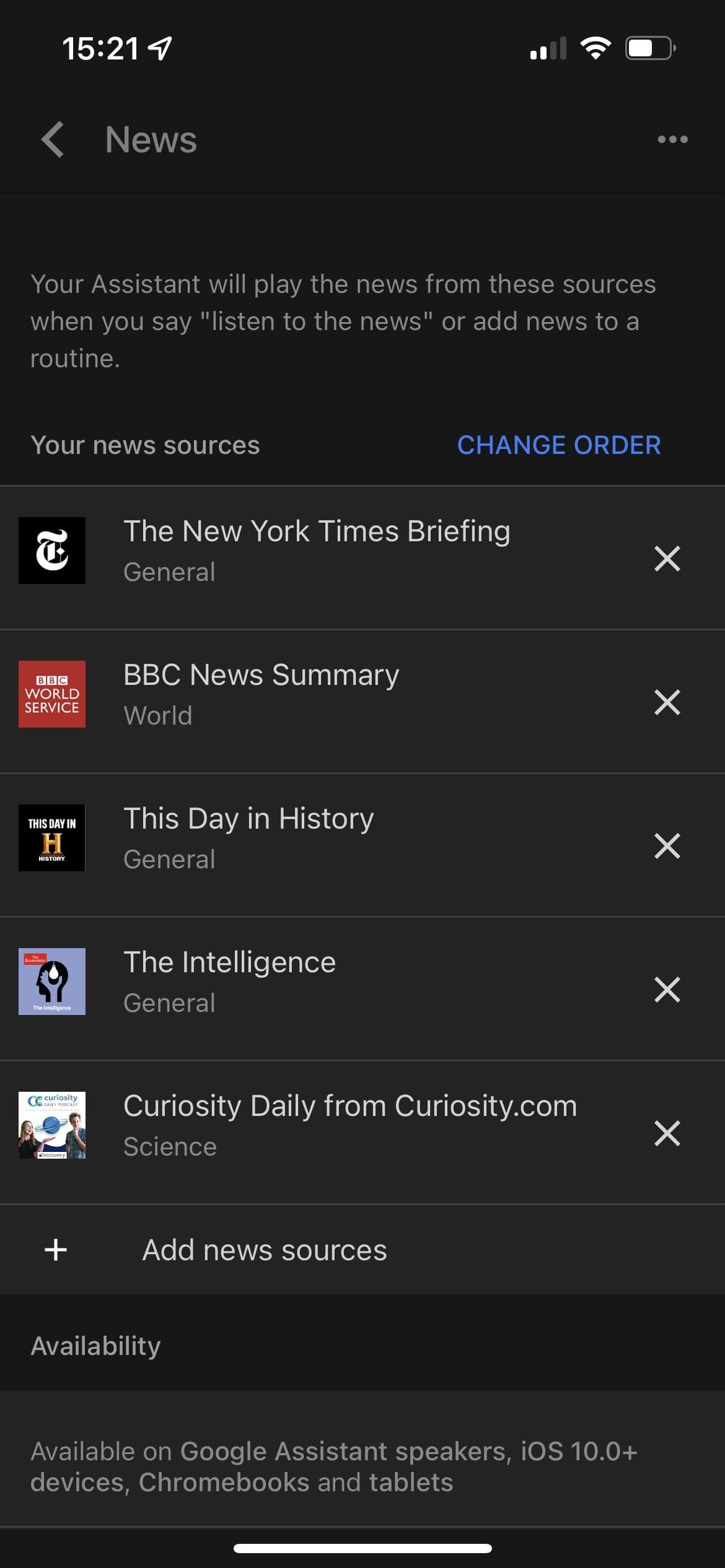The image is a screenshot of an iPhone in dark mode displaying the News app interface. In the upper left corner, the time reads 15:21 next to a navigation arrow pointing right. In the upper right corner, the status bar shows two out of four bars of cellular signal, a Wi-Fi signal icon, and a battery level about two-thirds full.

Prominently displayed is a notification stating: "Your assistant will play the news from these sources when you say 'listen to the news' or add news to a routine." This text appears in light gray on a black background.

Underneath, the selection of news sources is listed, showing five different options:
1. **The New York Times Briefing** – Icon: The iconic gothic 'T' on a black background. Category: General.
2. **BBC News Summary** – Icon: Classic red background with the white BBC logo and "World Service". Category: World.
3. **This Day in History** – Icon: The History Channel logo with "This Day in" at the top. Category: General.
4. **The Intelligence** – Icon: A silhouette in profile wearing headphones, reminiscent of the PBS logo. Category: General.
5. **Curiosity Daily from curiosity.com** – Icon: Two people with some partially visible blue text. Category: Science.

At the bottom of the screen, the app indicates categories listed for each source, along with a button to add more news sources. It specifies the availability of the News app on Google Assistant speakers, iOS 10.0+ devices, Chromebooks, and tablets.